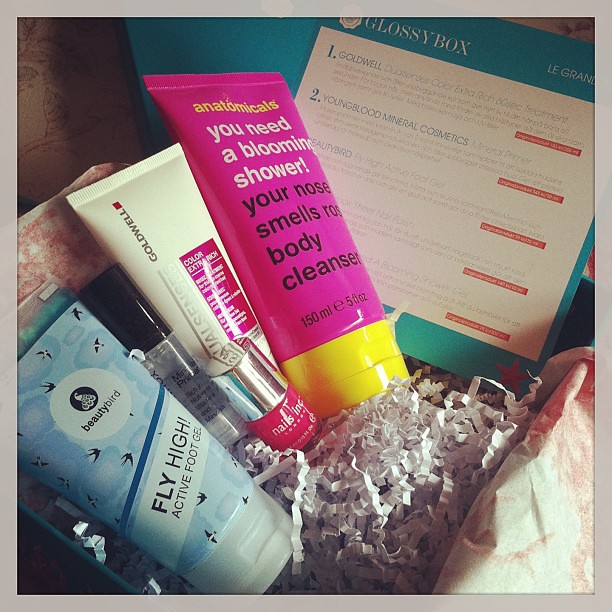This photograph captures a detailed close-up of a gift basket featuring a variety of personal care products. In the lower left-hand corner, there is a tube of Fly High Active Foot Gel by Beauty Bird, recognizable by its blue packaging adorned with small bird illustrations and a white cap. Adjacent to the foot gel is a bottle of bright pink nail polish with a chrome top. Next to the nail polish, there's a thin clear bottle filled with liquid and topped with a black cap, although its exact purpose is not mentioned. Moving further right, there is a tube labeled Goldwell Color Extra Rich, likely either a conditioner or shampoo, in off-white packaging. The largest item in the basket is an Anatomicals body cleanser, notable for its bright pink tube and yellow cap, with the label reading "You Need a Blooming Shower. Your Nose Smells Rose." All these items are neatly arranged in a basket filled with crinkled paper for padding. In the middle to the right, there's an insert with the title "Glossy Box," which provides a detailed explanation of each product included in the gift basket.